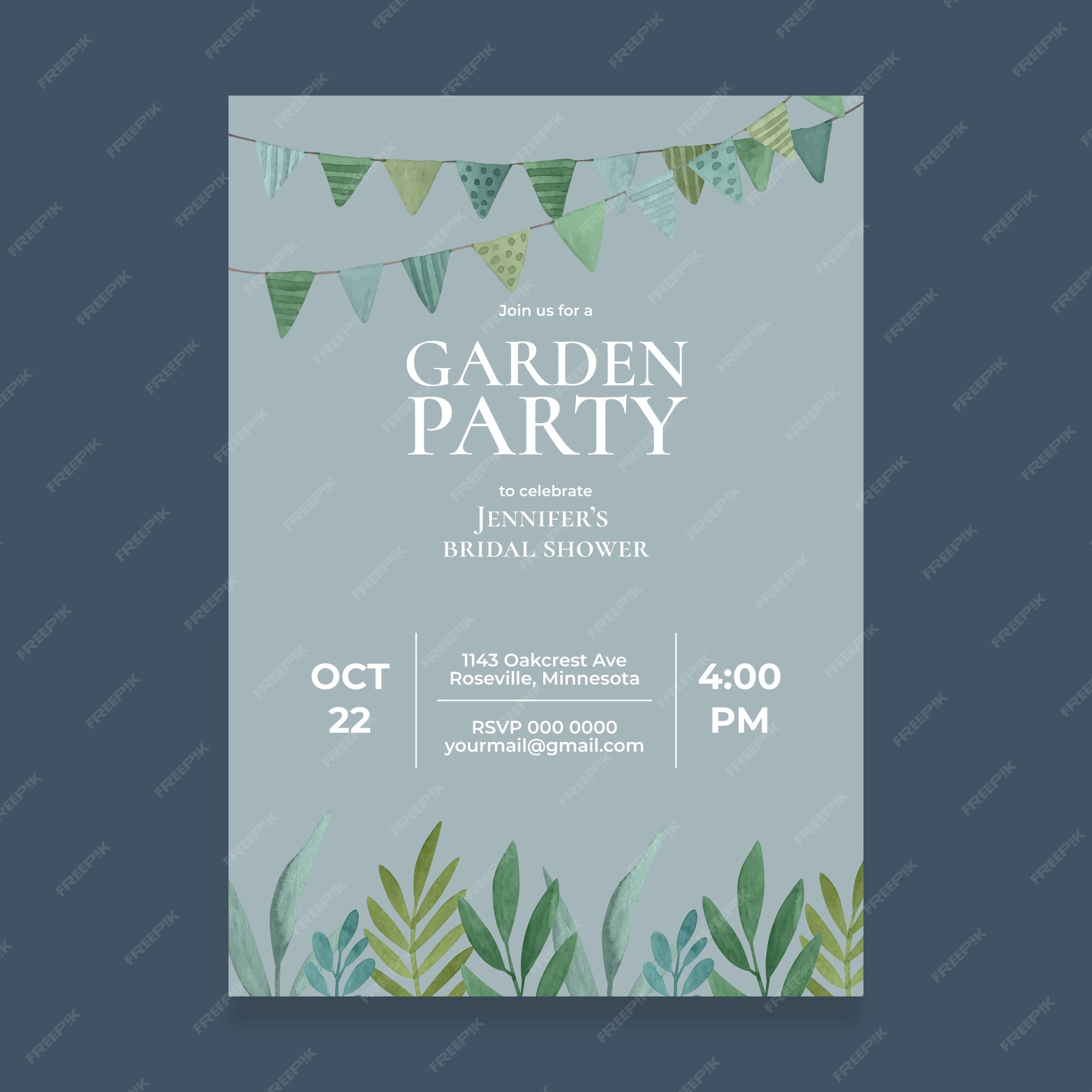This detailed image is a garden party invitation for Jennifer's bridal shower, showcasing a very light blue background with elegant white capital letters in the center. The top of the invitation features a colorful bunting banner strung across, displaying light green, light blue, pale yellow with blue polka dots, light tan, and light brown colored flags.

The main text reads:
- **GARDEN**
- **PARTY**
- **TO CELEBRATE**
- **JENNIFER'S**
- **BRIDAL SHOWER**

Further down, the invitation provides detailed event information:
- **DATE:** October 22
- **TIME:** 4:00 p.m.
- **ADDRESS:** 1143 Oakcrest Avenue, Roseville, Minnesota
- **RSVP:** 000-000-0000 / yourmail@gmail.com

The invitation is artistically decorated with drawings of wild leaves, including eucalyptus and ferns in various shades of green, blue, and mint at the bottom. This sample showcases a visually appealing design that highlights the upcoming celebratory garden party.